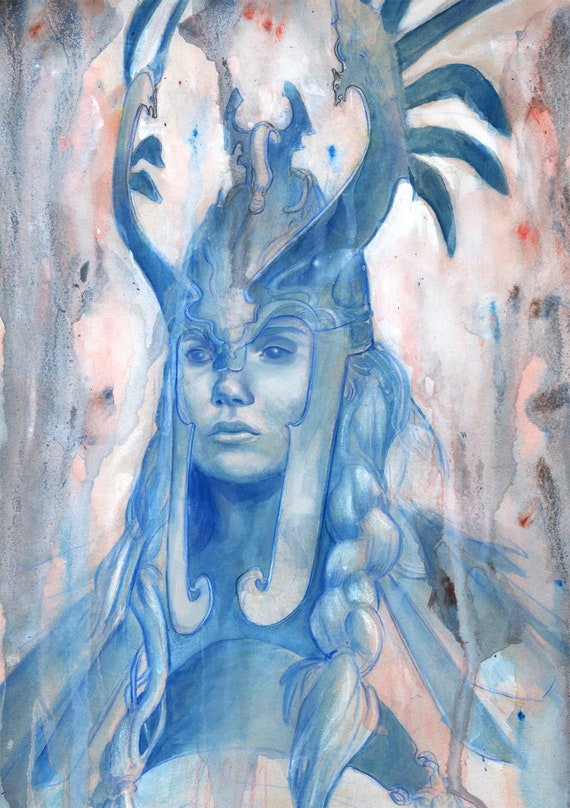This rectangular, possibly watercolor painting depicts a determined Nordic warrior woman, capturing her from her face to part of her upper body. The focal point of the artwork is her striking appearance: she wears a large helmet adorned with upward horn-like structures resembling feathers, which frame her face and extend down to her chest area. Her long hair, appearing blue in color and neatly braided into two locks, falls over her shoulders. The painting employs a predominantly blue palette for the warrior, contrasting with a softly muted background featuring pinks, peaches, and grays, suggesting the use of water to diffuse these colors. The composition emphasizes her warrior essence, blending the ethereal quality of watercolor with detailed pencil-like precision.